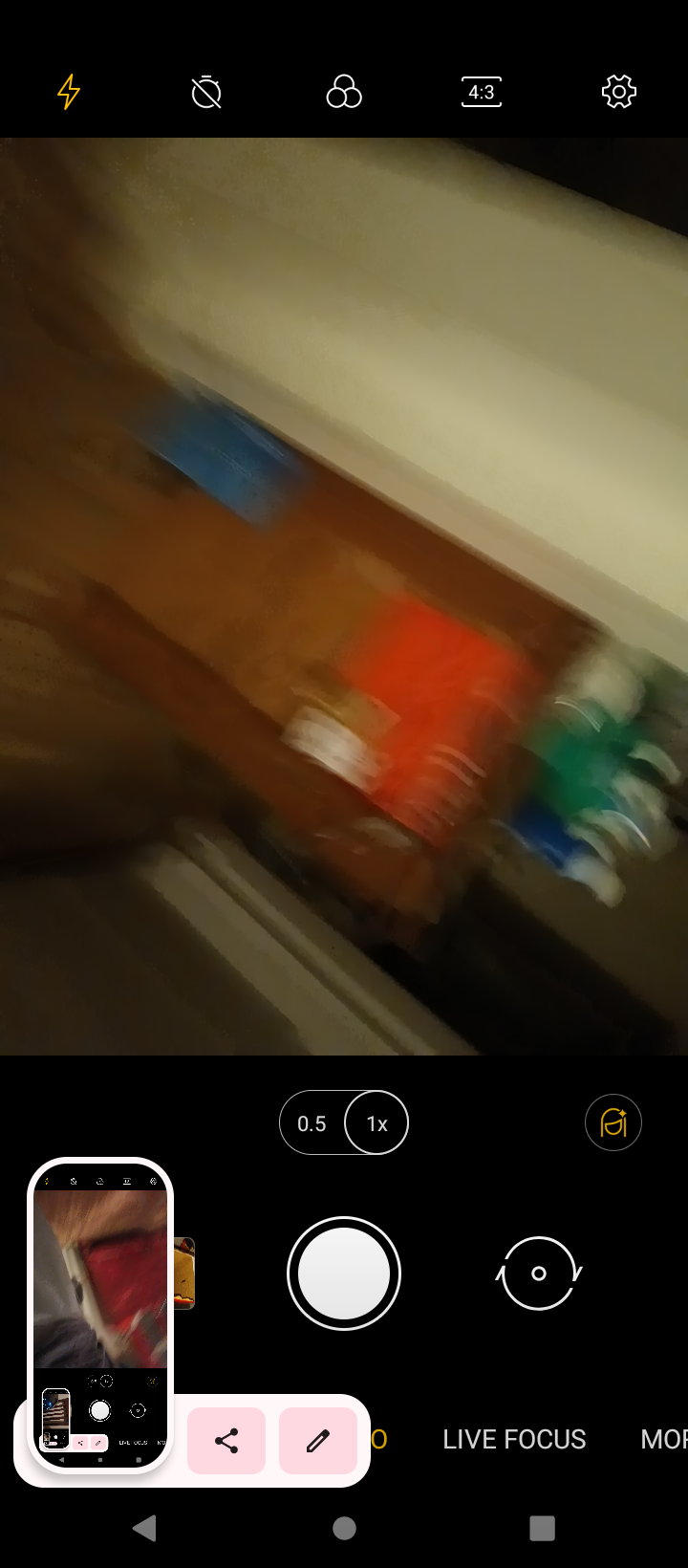A vertical aspect ratio image showing a blurry screenshot of someone using their smartphone's camera app. At the top, a black bar displays several icons representing different camera settings. The central viewfinder dominates the frame, showing an indistinct interior scene, possibly inside a home or building. Below, additional camera controls are visible, including the shutter button, a rotate button, and a zoom button. In the bottom left-hand corner, a screenshot dialog box indicates that a screenshot has just been captured, with options for sharing and editing the image through various buttons.